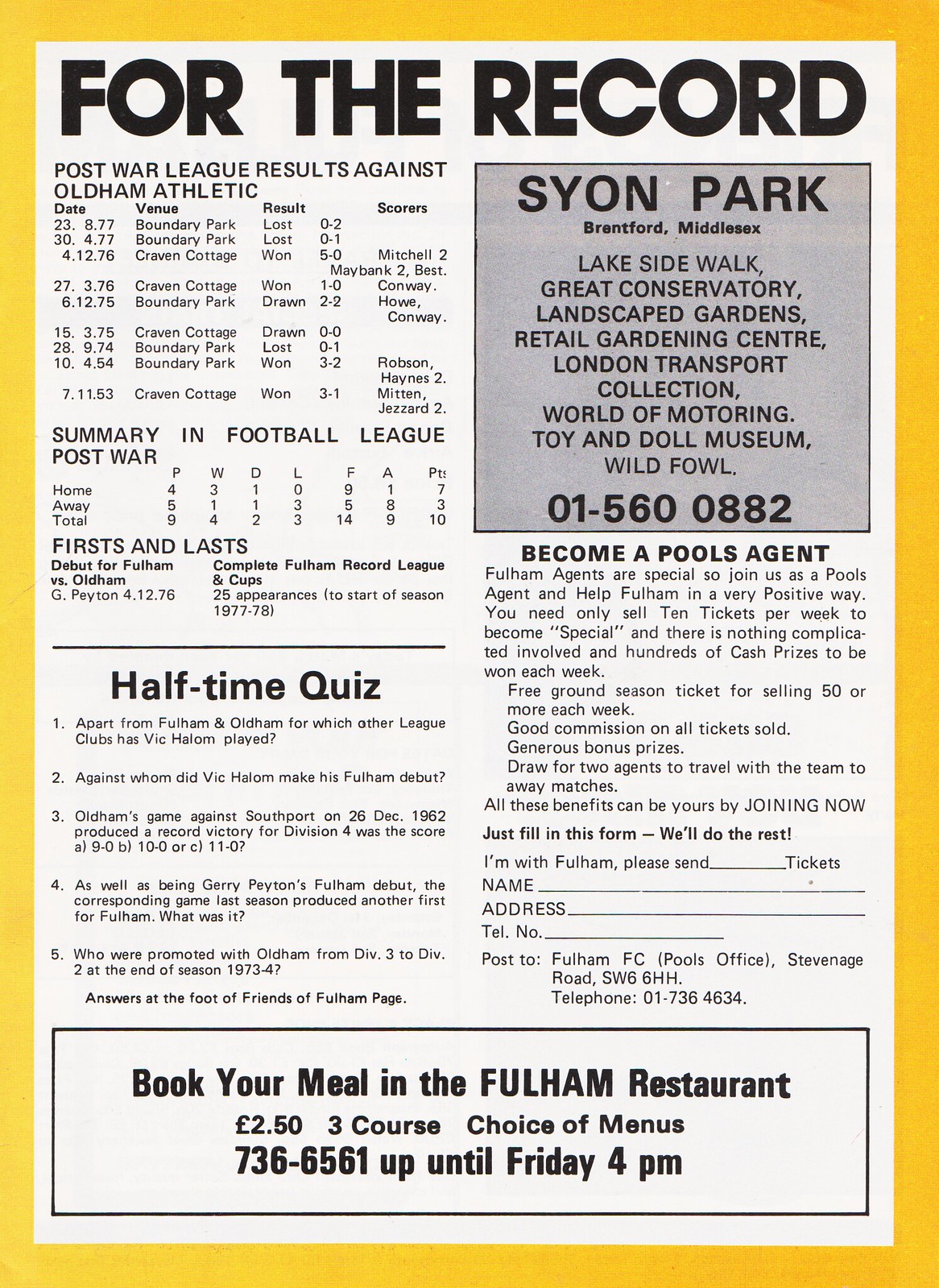The image depicts a scanned page from an old soccer magazine or program, presumably related to the Oldham Athletic Football Club. The page is framed by a yellow or golden border, with a white interior and black lettering. At the top, it prominently displays the heading "For the Record." The left column features several charts. The first one, labeled "Post-War League Results Against Oldham Athletic," lists the dates, venues, and scores of nine matches. Below this is a "Summary in Football League Post-War," detailing the figures for home, away, and total games: wins, losses, ties, points for, and points against. The third chart, titled "First and Last," is split into two sections, though the specific content is too small to read. Beneath these charts, separated by a black line, is a "Halftime Quiz" with five questions, the answers to which are not provided on this page. 

At the bottom of the left column is a horizontal advertisement for the Fulham Restaurant, offering a three-course meal for £2.50, and includes a booking phone number. The right column starts with a gray square highlighting "Scion Park" in bold letters, followed by a list of attractions such as Lakeside Walk, Great Conservatory, Landscaped Gardens, and more, along with a contact phone number. Under this is an ad encouraging readers to "Become a Pools Agent," detailing the benefits and requirements for selling tickets to support the club. There's a section for filling in the name, address, and telephone number to post to Fulham FC Pools Office, complete with contact information. The page is richly packed with historical soccer data, advertisements, and calls to action, presenting a vivid snapshot of the era's sporting culture.